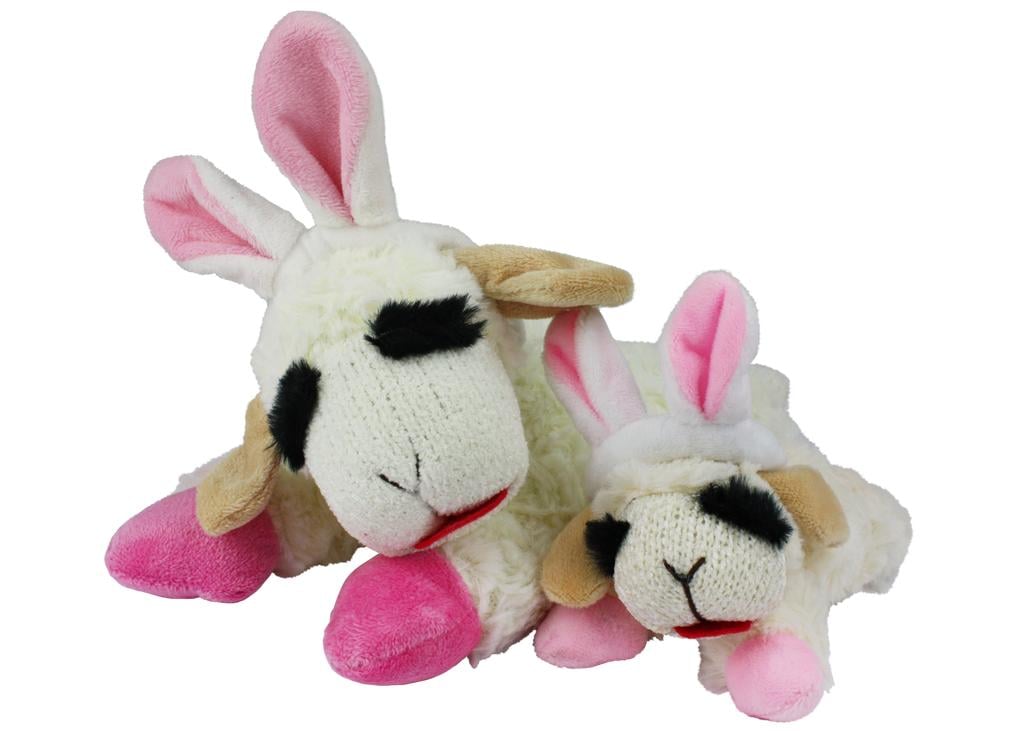The image depicts two stuffed bunnies, characterized by their wooly fabric bodies and crocheted faces, positioned lying down on their stomachs side by side, with the larger rabbit on the left and the smaller one on the right. Both bunnies feature a cream-colored body and have floppy light brown ears that hang down the sides of their heads, along with additional ears that stand upright with light pink insides, resembling typical bunny ears. Their eyes consist of black, furry rectangles, and they have pink nose stitches above red mouths. They are adorned with light fur atop their heads. The larger bunny's front paws are a darker pink, while the smaller bunny's paws are a lighter pink, both resembling pink velvet or knitted mitten toes.